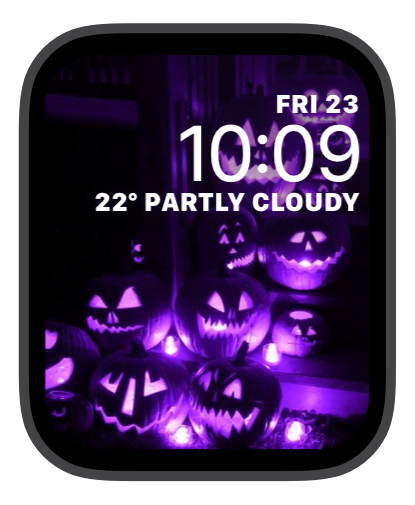The image showcases the face of an Apple Watch with a dark gray border and black-tinted glass around the screen. The screen displays various pieces of information against a visually intriguing background featuring a purple and black theme with jack-o'-lanterns emitting a purple glow. These jack-o'-lanterns are positioned on benches and add a unique, eerie atmosphere.

In the upper right corner of the screen, the date "Friday 23" is visible, presumably indicating Friday the 23rd. The time shown is 10:09, though the absence of an a.m. or p.m. designation leaves the exact time ambiguous. The weather is also displayed, indicating a temperature of 22 degrees and partly cloudy conditions, although it's unclear whether the temperature is in Fahrenheit or Celsius.

The overall presentation of the Apple Watch face combines functional time and weather details with a creatively themed background, making it visually appealing.